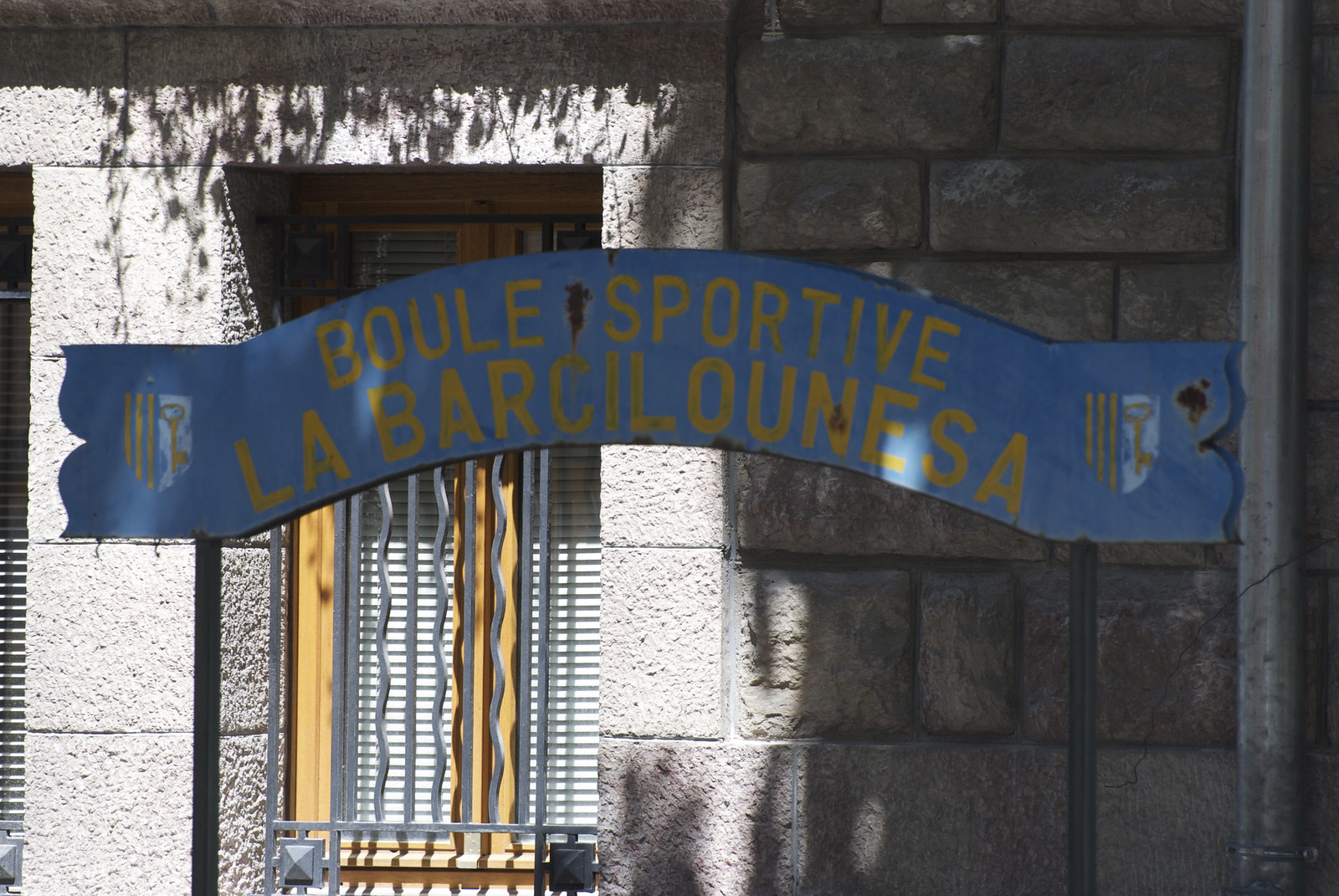The image depicts a gray brick building with large rectangular gray bricks. A noteworthy feature is the window on the building's side, protected by wavy metal bars, sectioned into squares in the top left, and bottom left and right corners. Adjacent to the window is a metal pipe, which appears to be part of a drainage system. The focal point of the image is a weathered blue banner, shaped like a half-circle ribbon. This banner spans horizontally above the window, almost reaching the metal pipe. It features yellow text that reads "Boul Sportive La Barcelonessa," with a notable amount of rust. Flanking both sides of the banner are shields, each displaying three yellow vertical lines on the left and a yellow key on a light blue background on the right, adding an emblematic touch to the worn banner.